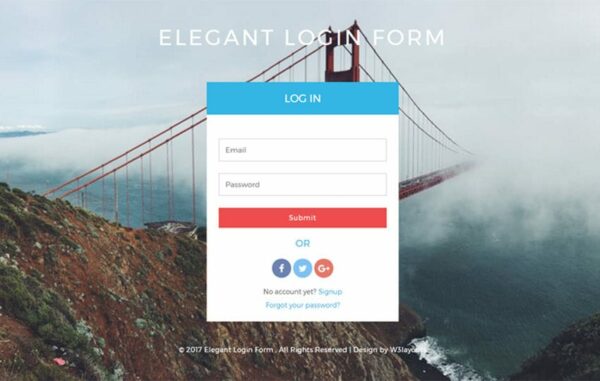The image displays a detailed and scenic login form set against a mountainous background. The top of the image prominently features the text "Elegant Login Form." 

### Background Description:
The background is dominated by a brown mountain with patches of green grass or other vegetation. Snow is visible on the mountain, hinting at a colder climate. The sky above is heavily clouded, creating an impression of either dense fog or an impending thunderstorm. Below the mountain, the outline of trees can be faintly seen through the mist or clouds. 

### Bridge and Structural Description:
In the foreground, possibly on a hillside, stands a large bridge. This bridge is characterized by two substantial red ropes or lines on either side, extending downwards with a series of vertical strings. At the highest point of the structure is a prominent metal piece from which the red ropes descend, curving down and to the right, disappearing into the fog, thereby obscuring the full extent of the bridge.

### Login Form Description:
Overlaying this picturesque scene is a rectangular login form. 
- The word "Login" is displayed at the very top in blue.
- Below it, fields for "Email" and "Password" are outlined in blue with white text.
- A red rectangular button labeled "Submit" is prominently placed below these fields.
- Under the submit button lies the text "Or," followed by the icons of Facebook, Google, and Twitter, indicating alternative login methods.
- At the bottom, the text "No account yet? Sign Up" is featured, with "Sign Up" in blue, contrasting the rest of the text in black.
- Additionally, "Forget your password?" is also in blue, offering users options for account recovery.

This meticulously described login form juxtaposed against the natural beauty of a mountainous landscape creates a visually appealing and functional user interface.